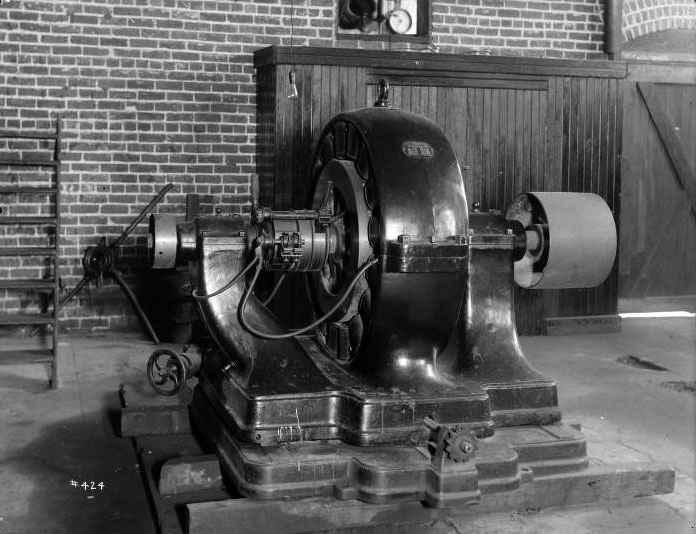This is a detailed black and white photograph depicting a large, antique piece of machinery prominently stationed in the center of an old factory setting. The backdrop features a brick wall on the left side, adjacent to a wooden wall on the right. Against the brick wall, a wooden ladder with eight steps leans halfway up. The central machinery includes a substantial, circular motor that resembles a large, shiny metal tire, with a solid metal shaft extending from both its sides. Each shaft supports a lathe-like instrument and is secured by two robust bars descending to a heavy metal base. The base rests on a concrete floor. In the background, partially concealed, is a wooden storage unit and what appears to be a barn door. Additionally, the bottom left corner of the image displays the number "#424". Various shades of gray accentuate the photograph’s vintage ambiance and the industrial elements within the indoor environment.